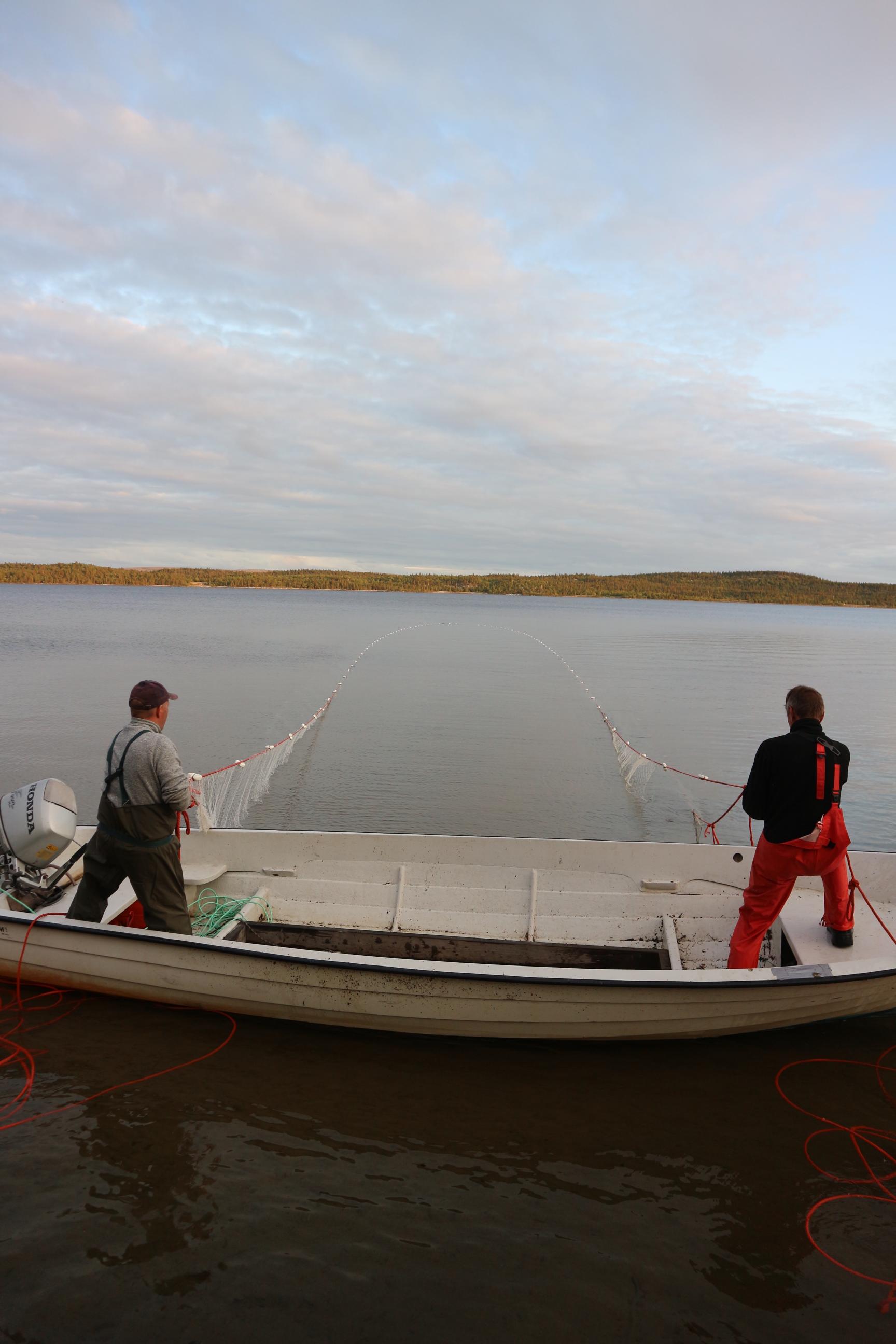In a vertically-oriented rectangle image, we see two men standing in a white, wooden boat set against the serene backdrop of a tranquil lake or river under a daytime sky. The sky occupies the upper third of the image, displaying a pale blue hue with thin, gray and peachy-colored clouds stretching across the horizon. In the distance, green land and smooth hills line the horizon, enhancing the tranquil ambiance of the scene.

The water beneath the boat is a dark grayish-blue, likely reflecting the sky above. The boat, which features a small motor on its left side, spans horizontally across the image. Standing at opposite ends of the boat with their backs to the camera, the two men are busy pulling up long white nets with red poles running through them. The nets, still partially submerged, show signs of being actively lifted from the water.

The man on the left is dressed in a dark baseball cap, a gray shirt, and dark green overalls or wader pants. His counterpart on the right is wearing a black shirt and striking red or orange overalls. Both men appear focused on their task of pulling in the nets, embodying the quiet diligence of a day's labor on the water. A small, unreadable red signature is located in the lower right corner of the image, adding a subtle artistic touch.